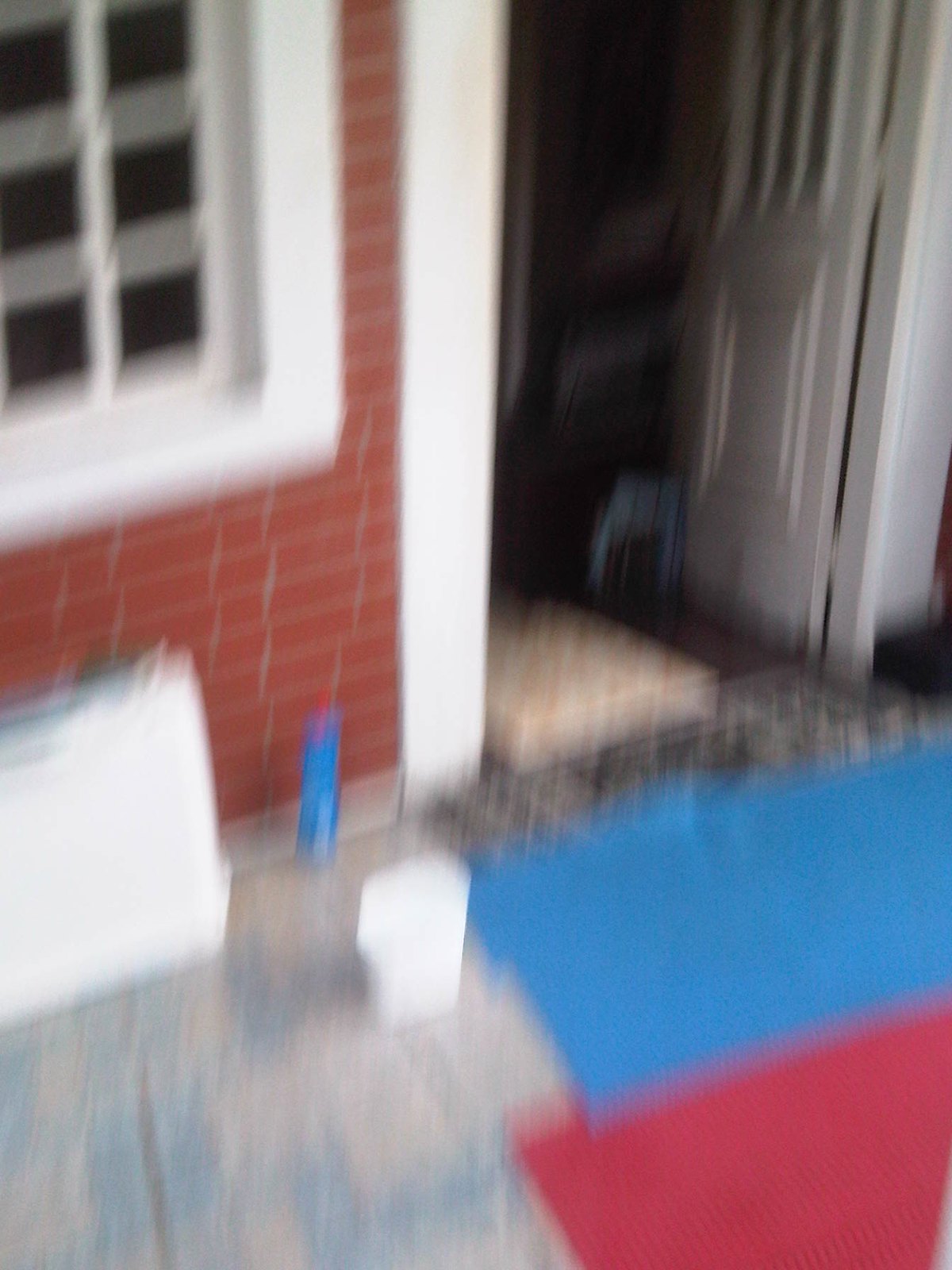A blurry photograph captures the exterior of a red brick house, possibly the back door, framed by large white panels. The white door, currently open, stands out against the brick, alongside a window featuring criss-cross wood detailing that divides it into small panes. The scene suggests some recent cleaning activity, evidenced by the presence of a blue bottle, potentially bleach, on the concrete floor which is slightly yellowed and tiled. Blue squiggly lines, possibly chalk smudges, are visible on the floor. Near the doorway, two pieces of fabric, one blue and one red, are spread out, resembling towels or rugs. Additional details include a large white object and a smaller white container near the entrance. Due to the photo's significant blurriness, these elements lack sharp clarity, contributing to an overall out-of-focus appearance.